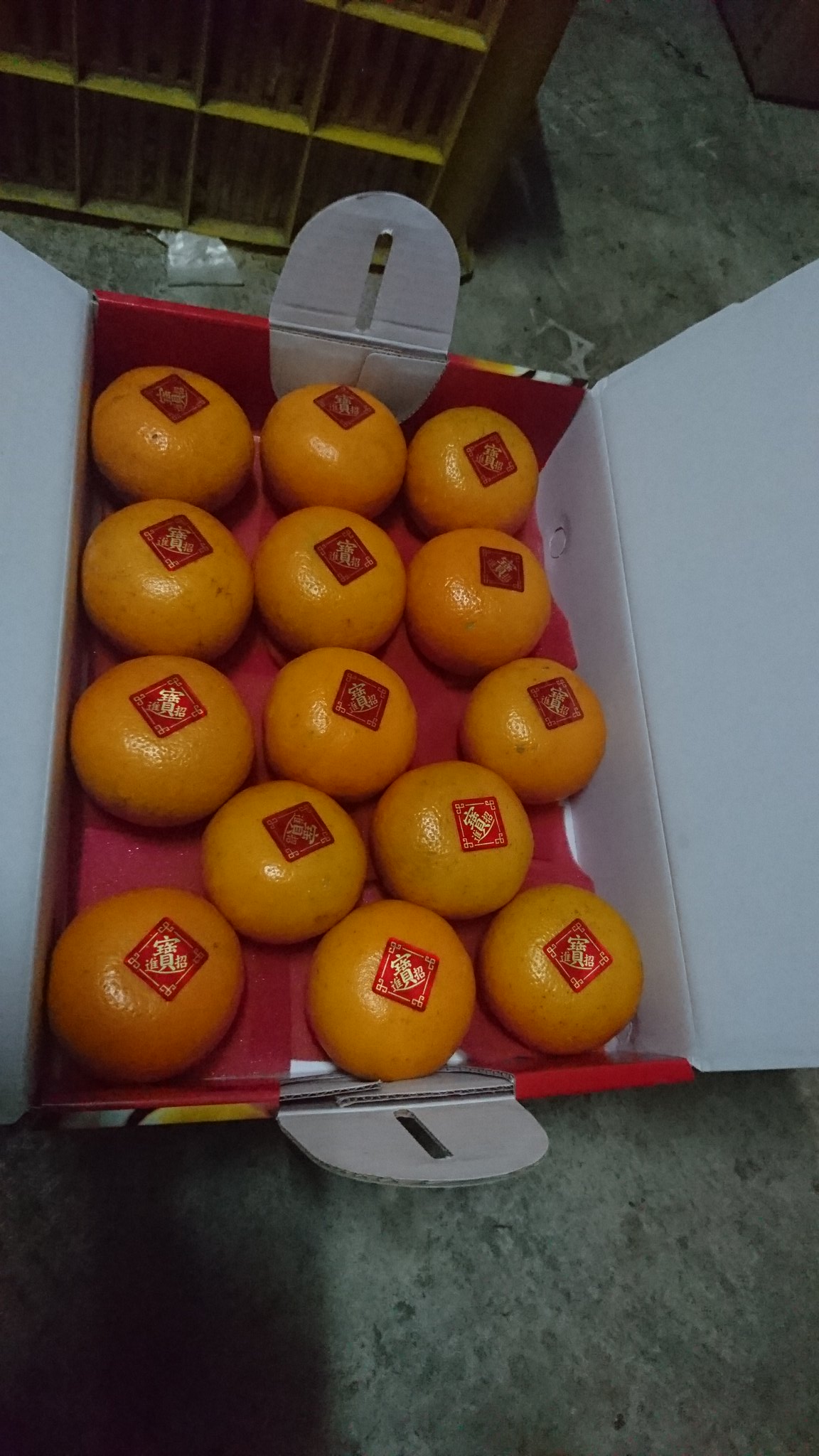This is a portrait-oriented color photograph of a white cardboard box, positioned on a mottled gray concrete floor, which is open to reveal 14 slightly flattened, uniform tangerines. Each tangerine has a distinctive red, diamond-shaped sticker with gold Chinese characters. The interior of the box is lined with red tissue paper, enhancing the festive appearance, possibly intended for an Asian holiday gift. The inside walls of the box are white, while the flaps that fold over are red on the inside. The image captures additional context: a green plastic crate with yellow centerpieces in the upper left corner, and a tan cardboard box in the upper right corner, suggesting the setting might be a warehouse or a storage area. Lighting is dim, causing some shadows on the floor.